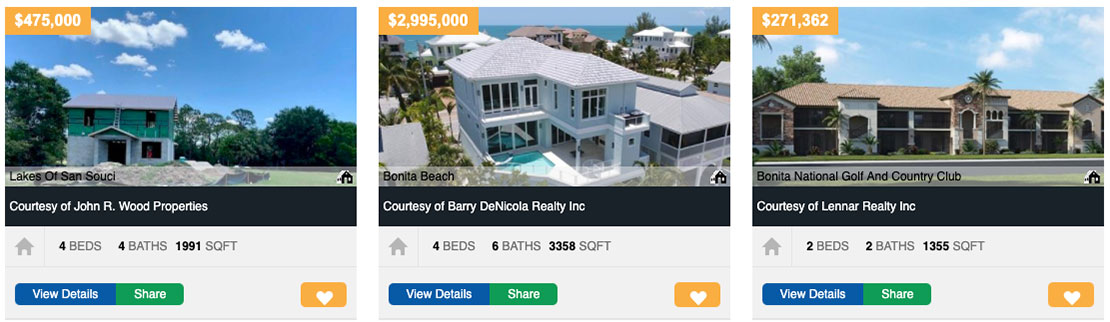**Detailed Descriptive Caption:**

The image showcases a segmented display of three property listings, resembling a user interface of either a mobile app or a desktop application, designed for a realty company or a platform such as Airbnb. Each segment is separated by small squares, highlighting individual properties.

1. **Lakes of Sanzuchi Property:**
   - **Visual Appearance:** The first segment features a picturesque house set in a sunny area, surrounded by lush trees and beneath a bright blue sky with a few scattered white clouds.
   - **Details:** Priced at $475,000, indicated by an orange rectangle at the top left corner.
   - **Additional Information:** Property details include a spacious layout of four bedrooms and four bathrooms within 1,891 square feet.
   - **Actions:** Below the image, there are interactive buttons - a blue "View Details" button and a green "Share" button, complemented by a rectangular heart button to save the property to a wishlist.
   - **Realtor Information:** Lakes of Sanzuchi, courtesy of John R. Wood Properties.

2. **Bonita Beach Property:**
   - **Visual Appearance:** The second segment showcases a substantial two-story house located in Bonita Beach.
   - **Details:** Listed under Barry DeNicola Realty Inc., this property boasts a significant size with four bedrooms, six bathrooms, and an expansive 3,358 square feet. It also features a swimming pool.
   - **Actions:** Similar to the first property, this segment has "View Details" and "Share" buttons below the image, along with a rectangular heart button for saving.
   - **Realtor Information:** Bonita Beach, courtesy of Barry DeNicola Realty Inc.

3. **Bonita National Golf and Country Club Property:**
   - **Visual Appearance:** The final segment displays a lengthy house with multiple column structures and surrounded by palm trees.
   - **Details:** Positioned within the Bonita National Golf and Country Club, this property includes two bedrooms, two bathrooms, and encompasses 1,355 square feet.
   - **Actions:** The interface is consistent with the previous segments, featuring "View Details" and "Share" buttons, along with a like/save heart button.
   - **Realtor Information:** Bonita National Golf and Country Club, courtesy of Lenar Realty Inc.

The entire image collectively presents a well-organized, visually appealing representation of different real estate listings with pertinent details and interactive features for potential buyers.